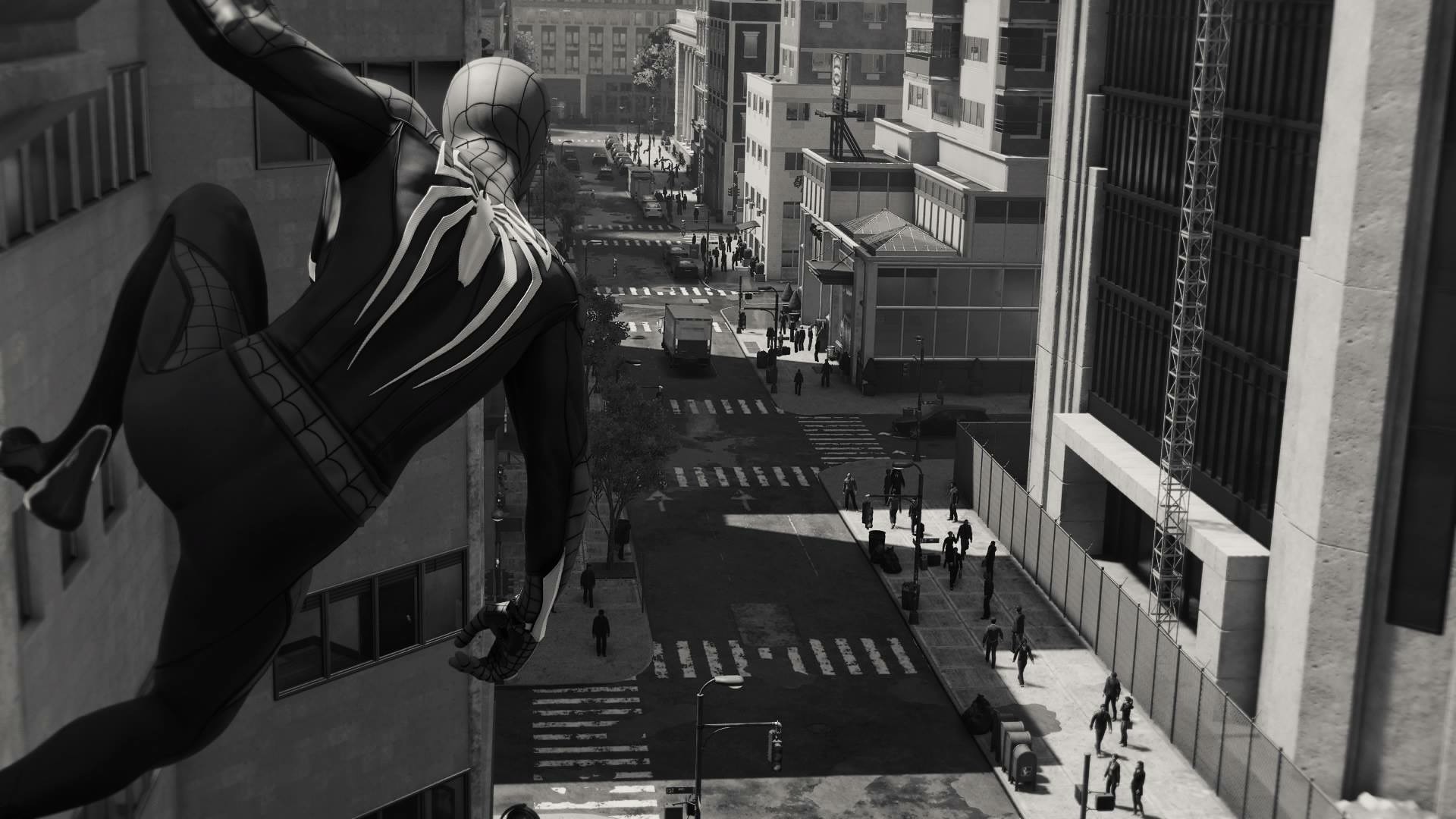This black and white image appears to be taken from a Spider-Man movie set or a video game still, capturing Spider-Man in his full suit hanging off the side of a tall building. Spider-Man is positioned on the left of the frame, his body suspended and his right hand hanging loosely as he looks down at the bustling city street below. The street runs through the center of the image, flanked by numerous tall buildings that cast shadows over the scene. 

Near the bottom right of the image, a construction fence encloses a segment of a building, featuring a prominent silver structure, possibly part of a crane or support system. A solitary box truck with a white box and black cab drives down the narrow road, which is dotted with around ten crosswalks. Crowds of people walk along the sidewalks on both sides of the street, appearing as black silhouettes against the brightness of daylight. Despite the monochrome palette, the image vividly conveys the contrast between light and shadow, emphasizing the city's architectural lines and dynamic street life below Spider-Man's vigil.